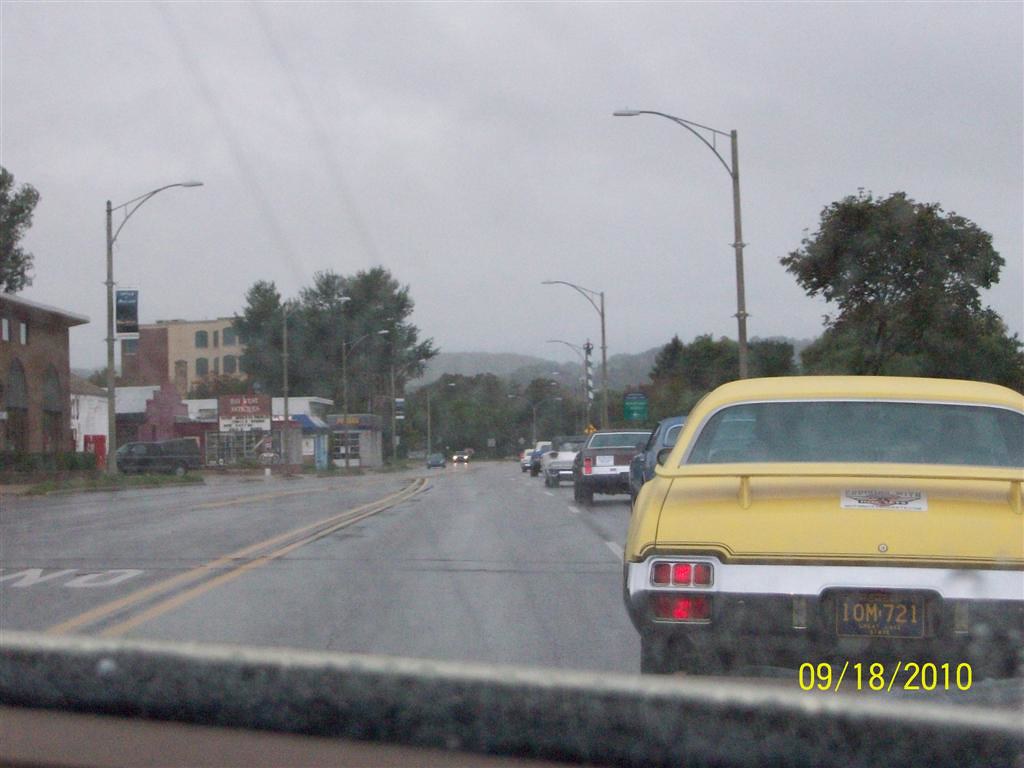The image, captured in landscape mode from within a vehicle—likely from the passenger side—displays a four-lane street scene from a dash cam on September 18, 2010, as indicated by the date stamp in the bottom right corner. The street is flanked by double yellow lines on the left and white dotted lines on the right, showcasing a lineup of vintage cars heading in the same direction. The closest car is a light yellow, old-timey vehicle, possibly a Mustang with a license plate reading "IOM.721" against a navy background. Ahead, there's a parade of five cars in varied colors—blue, black, white, and silver—all exhibiting distinctive classic styles, suggesting a procession of collector cars. The scene unfolds in a small town adorned with brick buildings to the left, possibly housing a mechanic shop, and other unidentifiable structures. Light posts and numerous trees line the road, with hills visible in the distance. The sky, grey and overcast, forebodes imminent rain, casting a gloomy ambiance over the otherwise vibrant parade of classic automobiles.